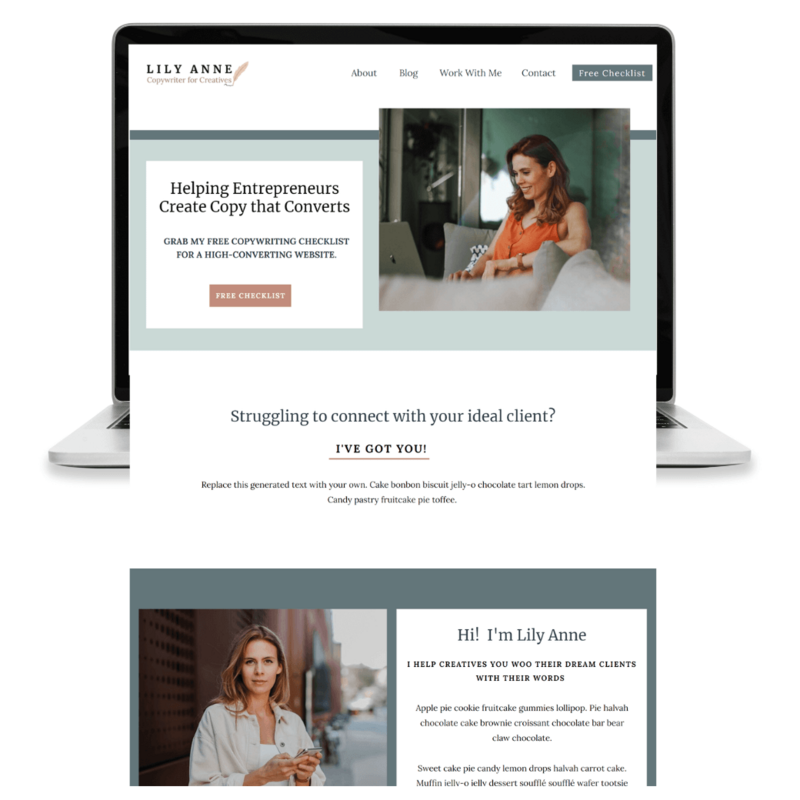The image showcases a web page displayed on the screen of an open notebook computer, creating a captivating 3D effect as the web page imagery extends downward beyond the laptop's frame. The web page has a white background complemented by two distinct shades of green: a pastel green and a deep olive green.

In the upper right portion of the web page, there is a picture of a woman with a warm smile, dressed in an orange sleeveless v-neck blouse. She is seated on a couch adorned with pale gray pillows. To the left of her image, within a white rectangular box with black text, reads: "Helping entrepreneurs create copy that converts. Grab my free copywriting checklist for a high converting website."